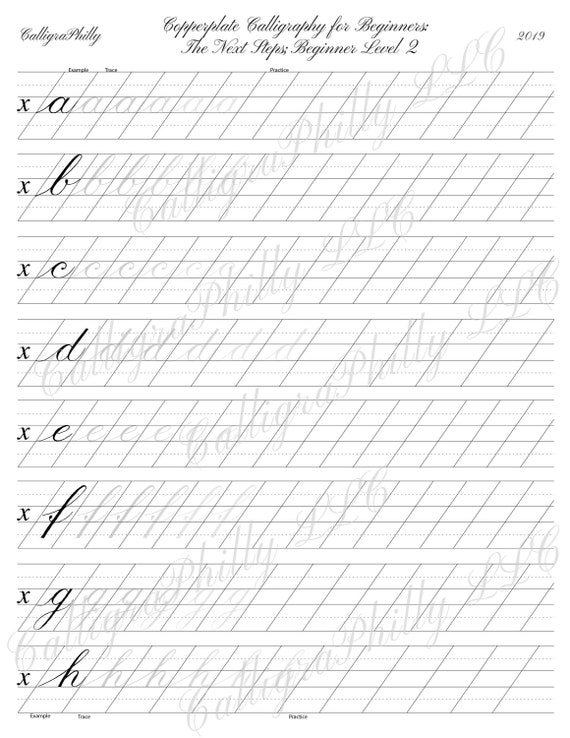The image shows a practice sheet for a calligraphy workshop titled "Calligraphy for Beginners: The Next Steps, Beginner Level 2." The sheet is dated 2019 and features rows of guidelines for practicing cursive letters. Each row comprises three practice lines designed to help learners master the flow of each letter. The guidelines for each line include two solid lines and a dotted middle line for spacing. Additionally, the practice lines are slanted from bottom left to top right to ensure the correct slant of the letters. The letters A to H are already printed on the page, becoming progressively lighter to almost translucent, allowing users to trace and practice each letter three times. Across the sheet is a watermark reading "Calligraphy Philly LLC."